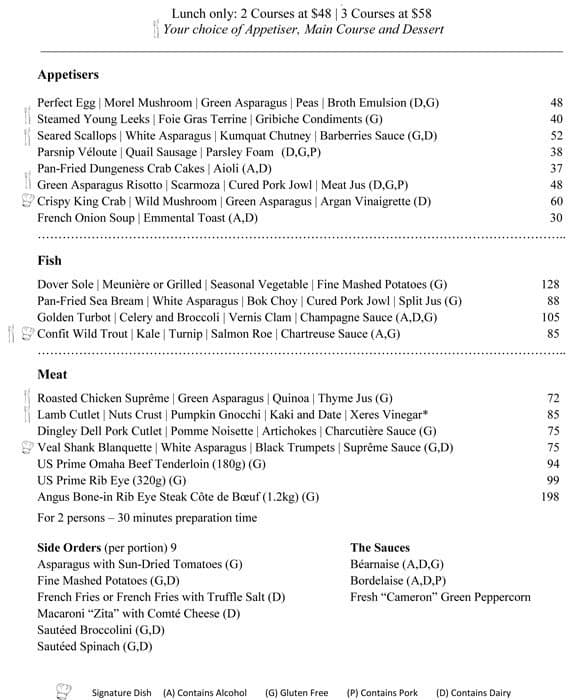The screenshot depicts a restaurant menu for lunch, detailing their two-course and three-course options priced at $48 and $58 respectively. The menu allows diners to choose an appetizer, main course, and dessert. 

Under the appetizers section, the options include:
- Perfect egg with mushrooms, asparagus, peas, and broth emulsion ($48)
- Pan-fried Dungeness crab cakes with aioli ($37)
- French onion soup with menthol toast ($30)

For the main courses:
- Fish dishes include Dover sole served with seasonal vegetables and mashed potatoes ($120), and confit wild trout with kale, turnip, and salmon roe, accompanied by a unique sauce ($85)
- Meat options feature roasted chicken supreme with green asparagus, quinoa, and thyme jus ($72), and a US prime ribeye priced at $99, which requires a 30-minute preparation time and is meant for two persons

The menu also includes side orders, such as broccoli and spinach, and various sauces.